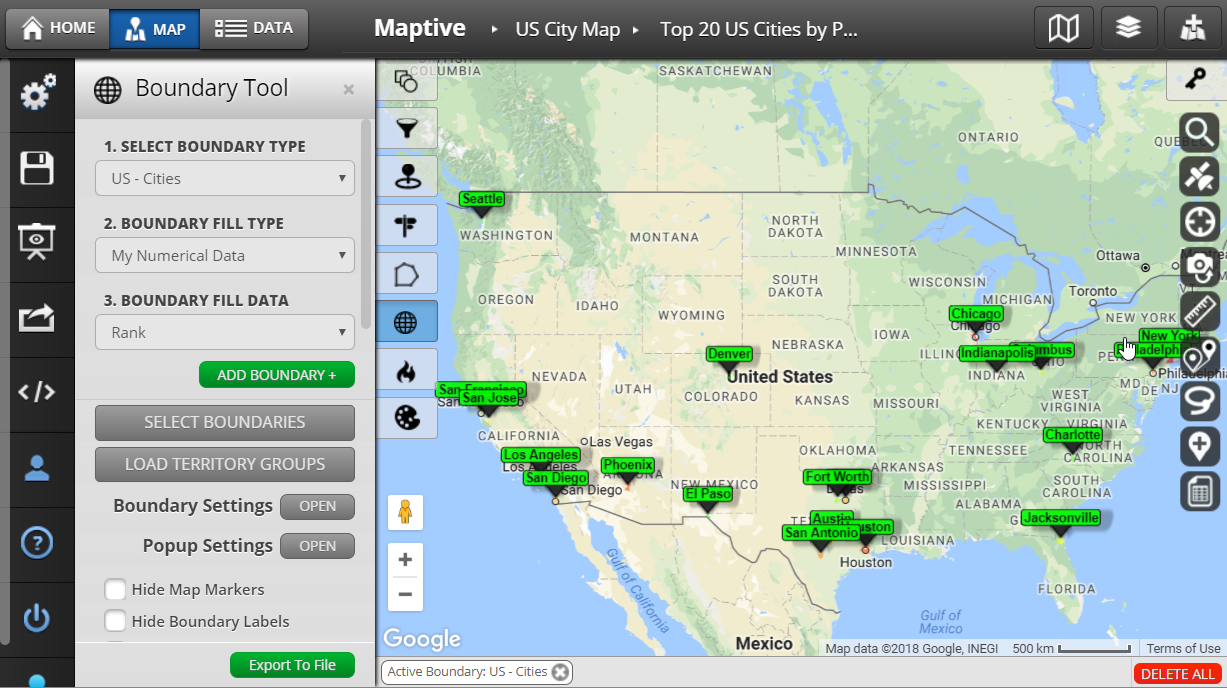This image is a detailed screenshot from the MAPTIV application, a digital map-rendering software tailored for creating and modifying maps. The interface features a prominent gray horizontal rectangle at the top, where the "Map" button is highlighted in blue. The application appears to focus on U.S. city maps, specifically highlighting the top 20 U.S. cities by population—although the word "population" is partially cut off.

Dominating the screen is a detailed map of the United States, showcasing various geographical features such as green areas indicating certain terrains, rivers, and locations of major cities. Major cities are marked with green rectangles accompanied by gray downward-facing triangles. The map also extends to include Mexico, providing a broader geographical context.

On the left side of the screen, a menu offers a variety of options for customizing the map. These options include "Boundary Types," "Boundary Fill Type," and "Boundary Fill Data," allowing users to select different types of boundaries. Below this menu, a sidebar includes settings for saving, taking screenshots, and other functionalities.

In the bottom right corner, an orange "Delete" button is prominently displayed. Additionally, a right-side menu features a legend in a square at the top, followed by a search bar and various icons that enable different functions related to map customization and location information. 

Overall, the interface is designed to be highly customizable and user-friendly, providing various tools for detailed map rendering.